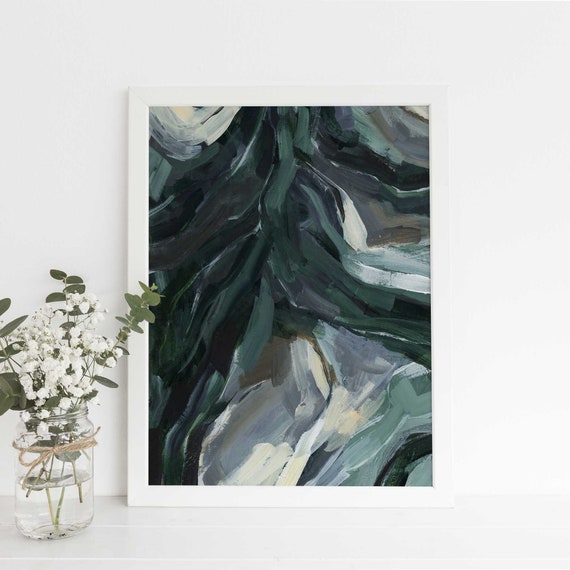In this scene, set against a white, cream-colored background, a detailed arrangement captures the eye. On the bottom left, a clear mason jar is positioned, filled halfway with water and adorned with a twine bow. Inside the mason jar, a tasteful arrangement of green leaves and small white flowers extends gracefully. Centrally staged, an abstract painting rests prominently. Featuring a white border, the canvas showcases an array of dark-toned colors including dark green, dark blue, cream, and white, applied in large, thick brushstrokes that create a flowing, almost river-like effect through the scene. The diverse palette includes grays, browns, and other dark hues, contributing to the mysterious and dynamic atmosphere of the abstract artwork.